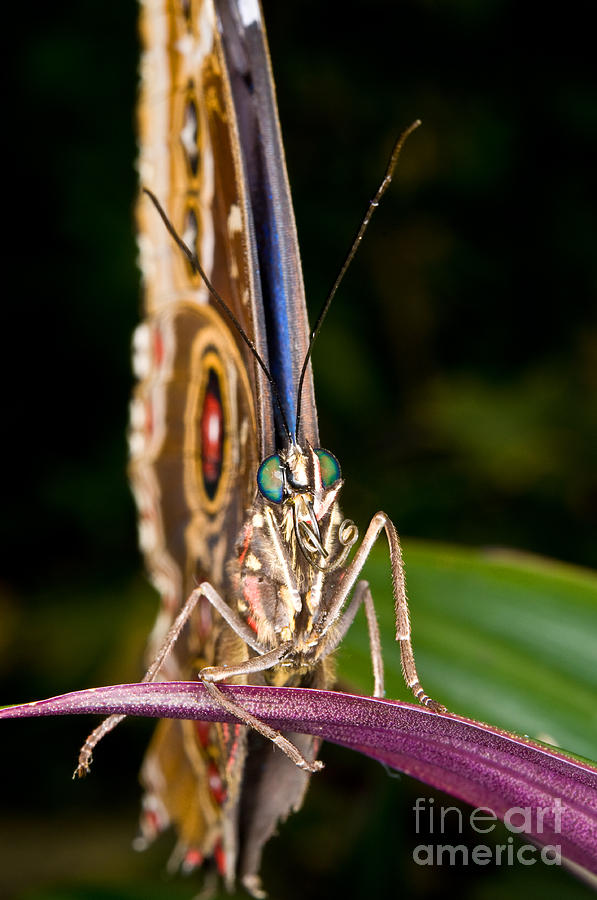This color photograph captures an extreme close-up of a butterfly perched on a purple leaf, a part of a vibrant plant. The butterfly faces the camera directly, its large, bright green eyes drawing immediate attention. Two black antennae extend upwards from its head. The butterfly clutches the leaf with its brown legs, which appear to shimmer with a golden hue under the lighting, and its body shares this brown-goldish tint, adorned with small hairs.

In the background, slightly to the right, lush green foliage is faintly visible, creating a contrasting backdrop for the subject. The butterfly's wings are folded back, with only the left wing partially visible. This wing displays a mesmerizing pattern of concentric circles in light brown, yellow, black, and red, all centered with white. Above these circles, smaller gold rings with black centers and white cores add intricate details. The outer edge of the wing features white spots set against a red background, completing the butterfly's striking appearance.